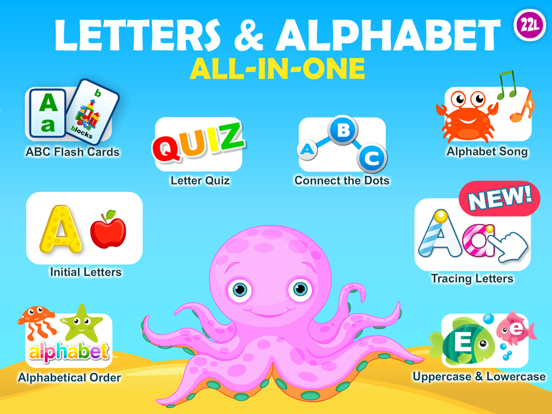A vibrant, child-friendly educational game screenshot showcases an engaging and colorful interface designed to teach children the alphabet. Dominated by the cheerful colors of blue, yellow, and a playful pink octopus, the background sets a lively tone for learning. At the top, the title "Letters and Alphabet All-in-One" is prominently displayed, with a circular element on the right-hand corner labeled "22L" in white text, outlined in purple.

The centerpiece features eight interactive icons representing different activities:
1. **ABC Flashcards** - Visual representations of flashcards to help recognize letters.
2. **Letter Quiz** - A colorful quiz with letters in red, orange, yellow, and green.
3. **Connect the Dots** - Engaging activity connecting alphabets in ABC sequence.
4. **Alphabet Song** - Illustrated with a crab and musical notes, making learning fun.
5. **Tracing Letters** - Features letters to trace with a hand icon, highlighted as a new game.
6. **Uppercase and Lowercase Letters** - Demonstrated by a big fish and a little fish for comparison.
7. **Initial Letters** - Depicted with an 'A' and an apple to associate letters with words.
8. **Alphabetical Order** - Encourages learning the sequence of the alphabet.

In the bottom center, the pink octopus icon adds a delightful touch to the educational game, inviting children to explore and enjoy various alphabet-related activities.